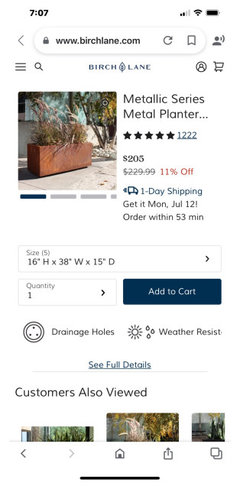The image is a vertically elongated screenshot of a smartphone screen, roughly three times taller than it is wide. At the top left corner, the time reads 7:07, and the top right corner displays full wireless signal, Wi-Fi signal, and a fully charged battery icon not plugged into a charger.

Just beneath this status bar, there's an address bar indicating the website being visited, "birchlane.com," with a padlock icon on the left signifying a secure connection. Adjacent to the address bar are buttons for reloading the page and opening a new tab.

Below the address bar, the website's navigation bar appears. On the far left are three horizontal lines symbolizing the menu, followed by a magnifying glass icon for search. The site's name, "Birchlane," is displayed in dark blue letters with a vertical leaf logo situated between "Birch" and "lane." To the right of the site’s name, there is a circle icon depicting a user, and next to it, a shopping cart icon.

The main content of the webpage shows a detailed view of a product. The featured item is a brown metallic planter, placed outdoors on a grey sidewalk block with some vegetation planted in it. To the right of the product image, there is a description: "Metallic Series Metal Planter," which is rated 5 stars based on 1,222 reviews. The current price listed is $205, with the previous price of $229.99 crossed out, indicating a discount. In red text next to the old price, it states "11% off." Below the price information, there is an icon of a truck followed by the text "One day shipping."